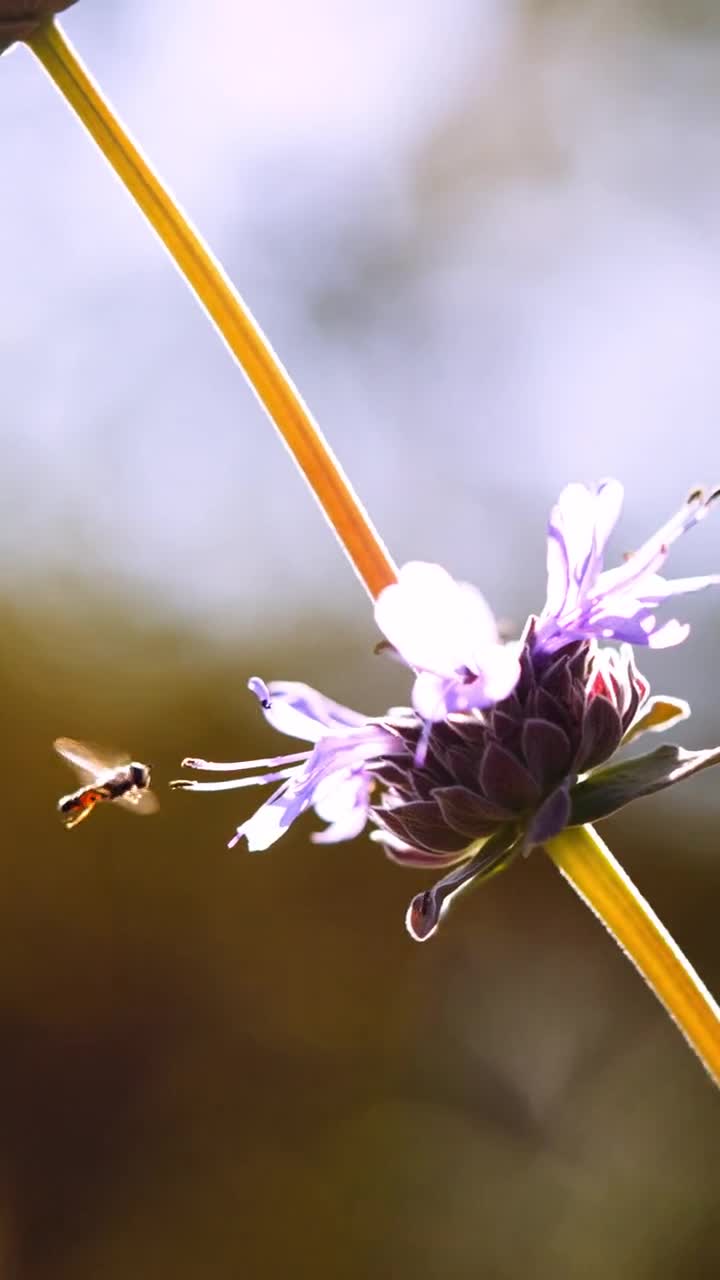This close-up, color photograph captures a stunning purple flower with intricate details and a bee in mid-flight approaching it. The flower's petals are a blend of dark purple at the base, transitioning to lighter purple and white at the tips, accented with tiny black tips. It is supported by a long, yellow-orange stem that curves diagonally from the lower right to the upper left of the image. Another similar stem extends parallel, disappearing out of the frame. The bee, positioned to the left of the flower, appears to be frozen in motion, its wings a blur, indicating rapid movement as it approaches for nectar or pollen. The background is entirely out of focus, composed of indistinct greenery and hints of blue sky, enhancing the prominence of the flower and the bee. The overall lighting suggests sunlight filtering from above, adding a natural glow to the scene, while the absence of any man-made structures or additional flora centers attention on this singular, captivating moment in nature.